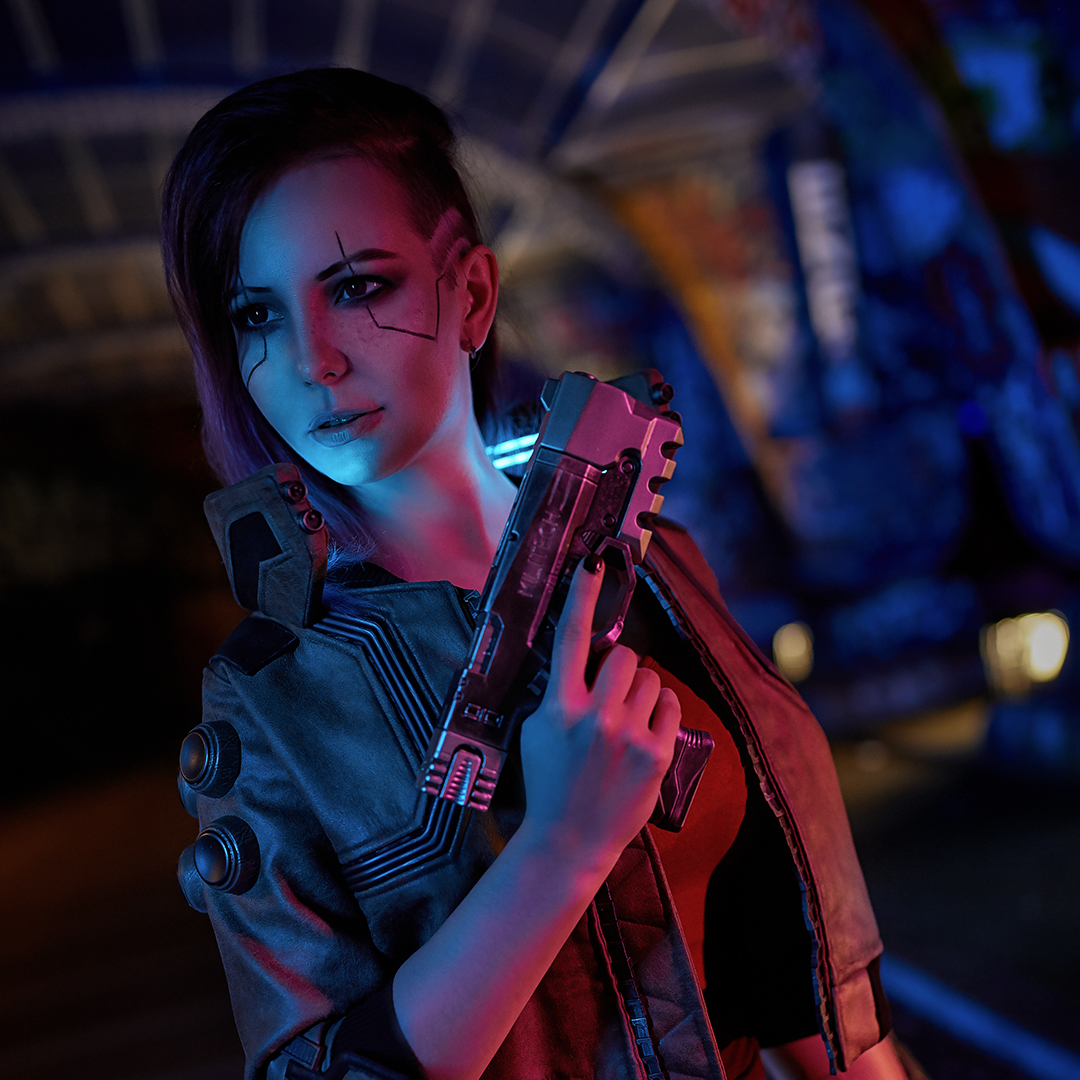The image depicts a female character who exudes a distinctly futuristic vibe, likely inspired by or from a game similar to Cyberpunk. Dominating the frame, she holds a large, bulky silver gun with black accents in her right hand. She is characterized by her striking dark purplish-brown hair, which features a stylishly shaved side adorned with lines. Her face is marked by a series of black, crooked lines running from her eyes to her ears, giving her an appearance of cracked skin or cybernetic modifications. Her piercing brown eyes and slightly parted lips offer a glimpse into her resolute demeanor.

She wears a short black jacket that ends at her forearms, paired with a red undershirt, adding to her sleek and elegant appearance. Black nail polish highlights her grip on the weapon, and her posture conveys a sense of confidence and elegance, although the weapon looks cumbersome. The jacket itself appears to feature LED lights around the neck area, further emphasizing the futuristic theme.

Behind her, the background is out of focus but hints at a dark, possibly underground environment, with faint lights casting minimal illumination on what appears to be spray-painted walls. The entire scene has a dimly lit ambiance, enhancing the mysterious and advanced setting of the image.